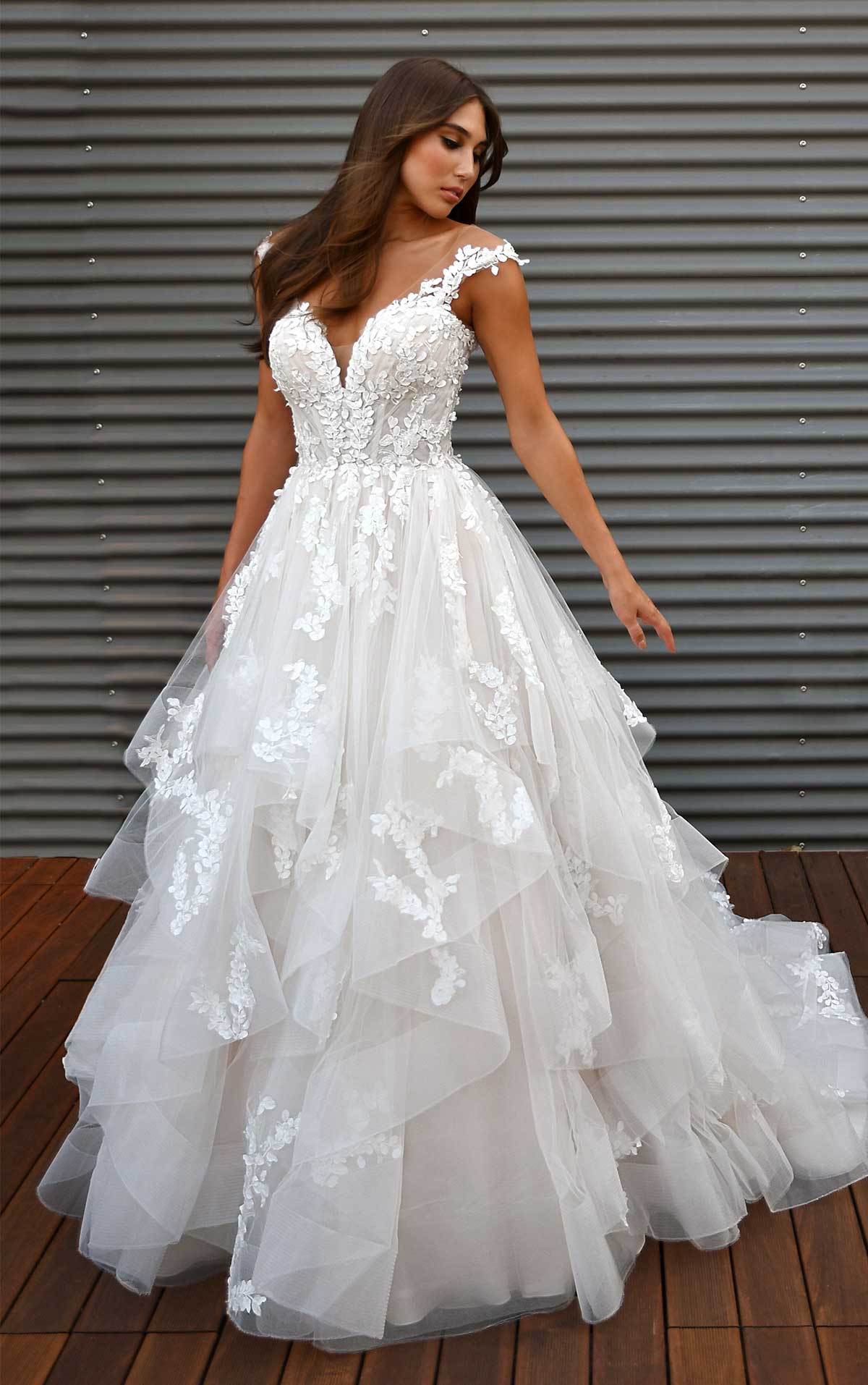In this detailed photo, a Caucasian brunette woman with long, straight hair, slightly curled at the front, is modeling a stunning wedding dress. She has a slight tan and is captured looking towards her left, with her chin directed to the side. Her left arm is elegantly outstretched around five o'clock, while her right hand is subtly hidden behind the elaborate gown. 

The wedding dress itself is a masterpiece, featuring delicate, tank-top-type sleeves adorned with floral lace that complement the deep-cut V bodice. The bodice is intricately designed with floral patterns that subtly transition into the layers below. The lower part of the dress is voluminous and fluffy, composed of asymmetric, lace ruffles and layers, and finishes with a flowing train that enhances the gown's grandeur. 

She is standing on a dark, tannish hardwood floor that adds warmth to the scene. The background is a textured gray wall, possibly a closed warehouse gate or shades, which is screwed on both sides, providing a stark contrast to the elegance of the bridal ensemble. The combined elements of the photo create a captivating image of bridal elegance and beauty.